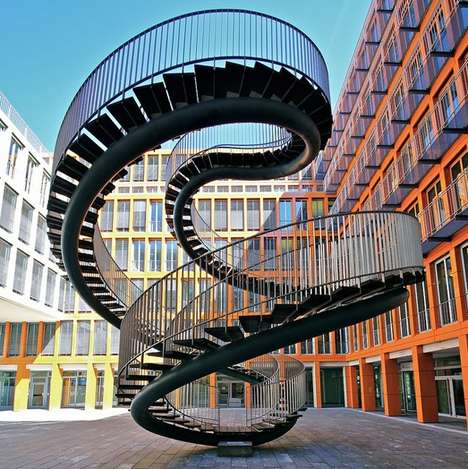The image features a large, freestanding spiral staircase positioned directly in the center, made from dark gray to black material, with a matching black railing. This staircase, resembling a twirled-up snake, loops around itself, seemingly leading nowhere and anchored only at its base to the stone brick floor. Surrounding this central staircase are multi-story buildings: an orange one on the right, a yellow one behind, and another yellow one on the left. These buildings are adorned with numerous windows. In the background, a light blue sky appears in the upper left corner, adding a touch of color to the scene. The setting suggests an outdoor courtyard or display yard, possibly within the artistic confines of a park or a residential area, giving the entire image an architectural and somewhat surreal feel.